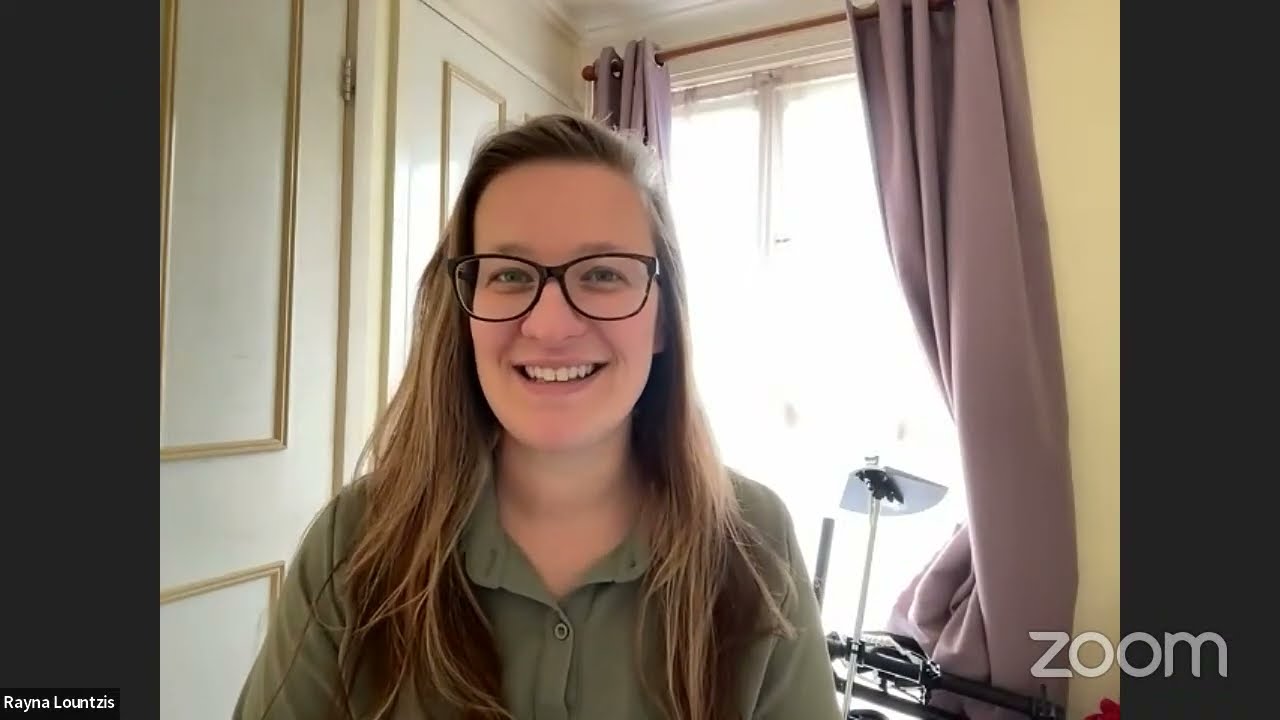This is a detailed screenshot of a Zoom call featuring a woman named Reyna Launtzis. You can identify the platform by the Zoom logo in the lower right and Reyna's name in the lower left, both set against black rectangles framing the image. Reyna has long, dirty blonde hair worn down and is smiling warmly. She is wearing thick black-rimmed glasses and a long-sleeve olive green button-down shirt. Reyna appears to be sitting down in a room, possibly a dining room or bedroom, bathed in natural daylight. Behind her to the right is a white wall with gold trim that frames a doorway or closet opening. An open window positioned behind her to the left allows abundant sunlight to flood in, though the window itself is closed. The light purple drapes are pulled apart and hang on a dark rod, bringing a softness to the scene. A lamp, situated on a black ledge next to the window, adds to the cozy ambiance. This carefully organized backdrop coupled with Reyna's engaging demeanor make for a well-composed and pleasant screenshot.